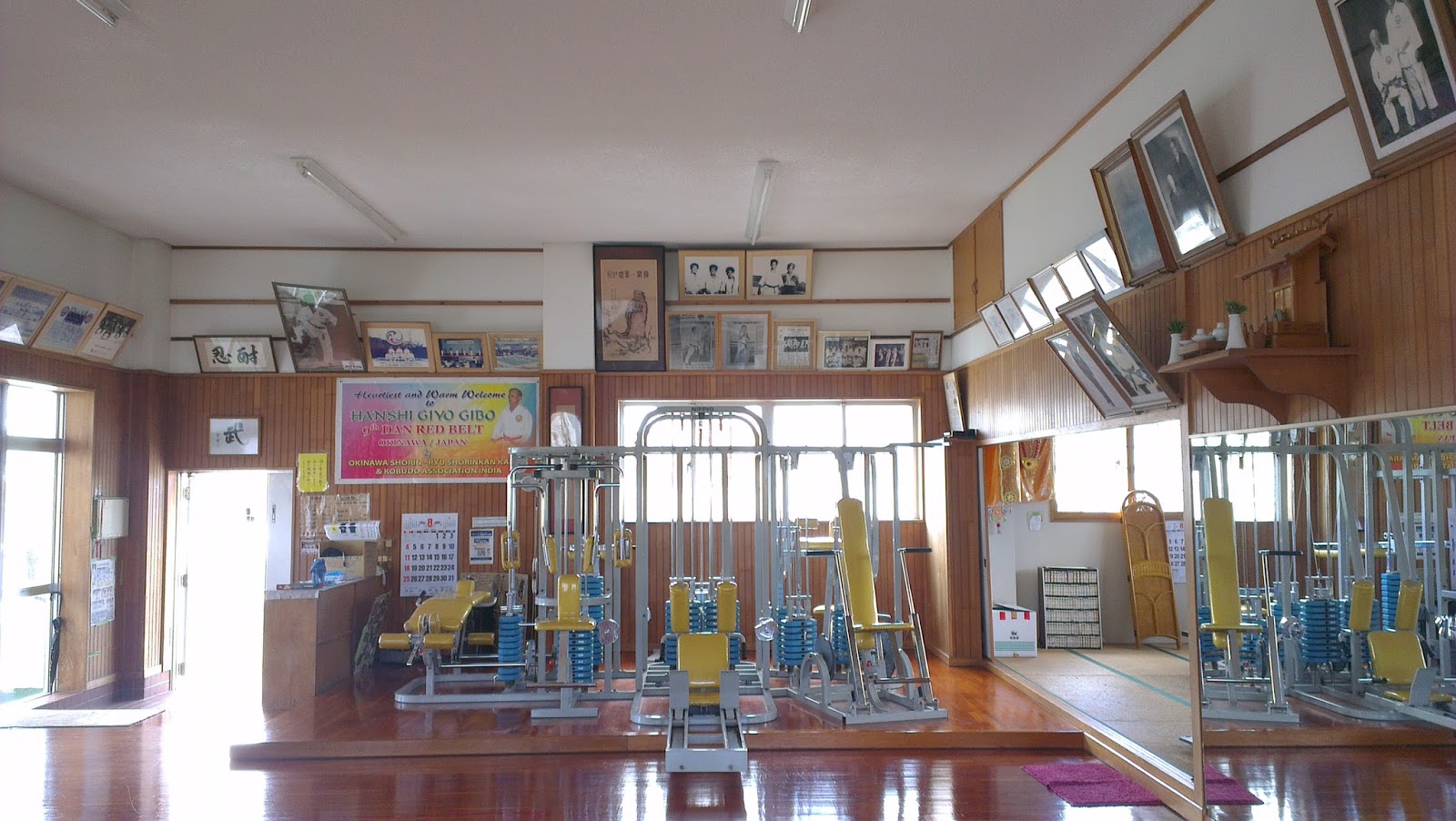This image captures a well-lit, indoor martial arts studio that doubles as a gym. The room is divided into two main areas: a primary gym section with a light brown wooden floor and a secondary raised room with white wood flooring accented with blue stripes. The gym equipment features benches and weights in shades of pale yellow and light blue, arranged on a wooden platform. A pink mat is noticeable in one corner.

The walls are adorned with various framed pictures and artwork. There are images of people in martial arts uniforms receiving awards, as well as portraits, black-and-white photos, and newspaper articles. Some framed art includes Chinese characters, and prominently displayed is a colorful banner that reads, "Welcome to Hanshi Gyo Gibo, 9th Dan Red Belt," referencing Japan and Okinawa.

Additional details include a door on the left side of the room with framed art above it, a counter with a calendar to its right, and several boxes against one wall. The studio is filled with natural light from numerous floor-to-ceiling windows, contributing to the overall clean and shiny appearance of the space. The ambiance is bright and welcoming, ideal for both martial arts training and general workouts.